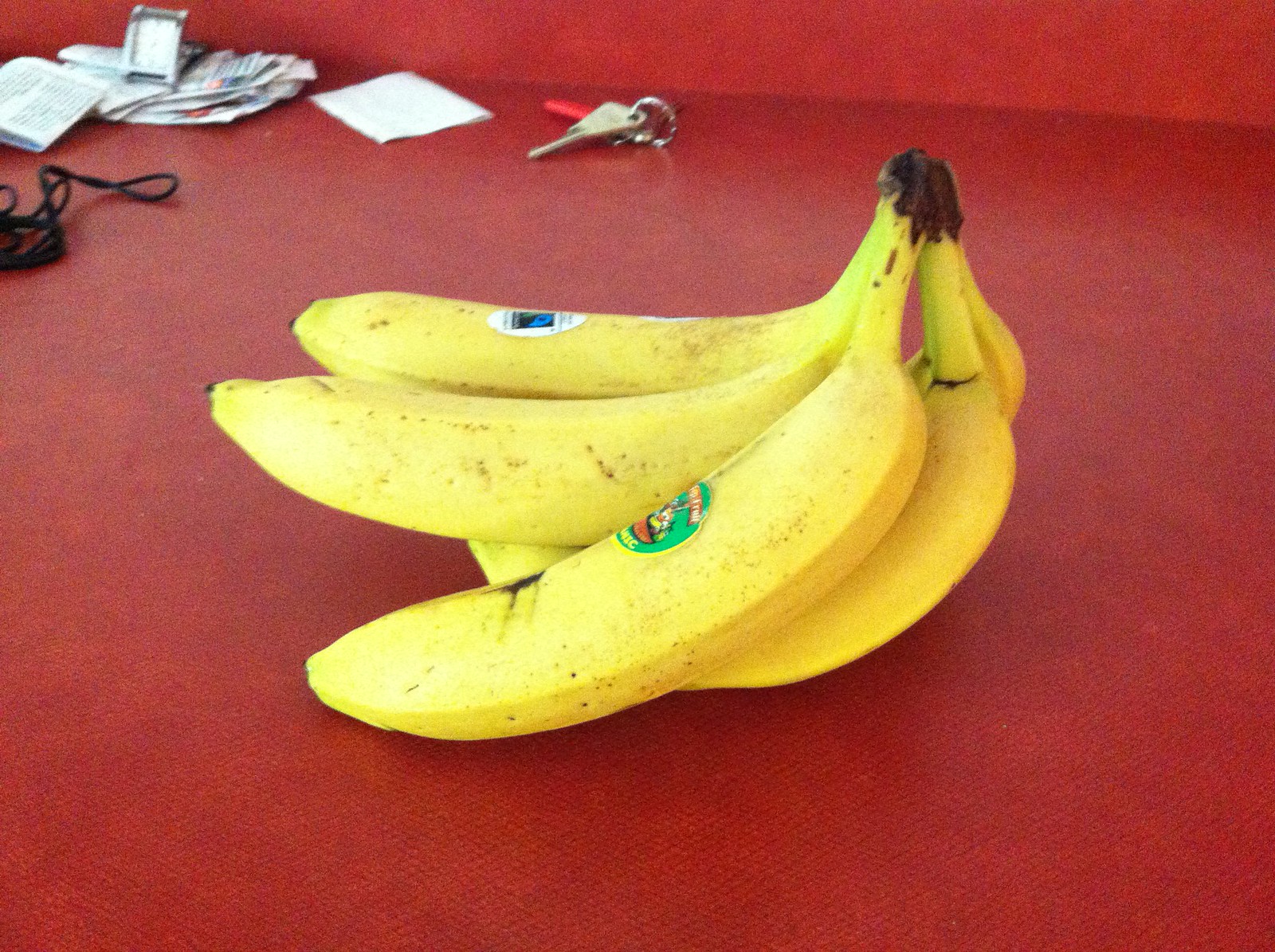In this striking image, the background is a vivid, solid red that extends to encompass the floor, the table, and the wall, delineated by a prominent line where the floor meets the wall. On the red table at the back, a set of keys with a red keychain lies next to what appears to be a white napkin, possibly from a restaurant. To the left of the napkin sits a small pile of newspapers or paper stack, adorned with printed text. At the forefront of this stack, a black wire or electronic cable subtly curves into view. Dominating the center of the image is a vibrant bunch of five ripe, yellow bananas. The trio of bananas on the left show natural brown speckles, while distinct stickers adorn the fruit – a green sticker prominently marks the front banana, and a contrasting blue and white sticker is seen on the leftmost banana. The meticulous arrangement of everyday objects against the uniform red backdrop creates a visually compelling and detailed composition.